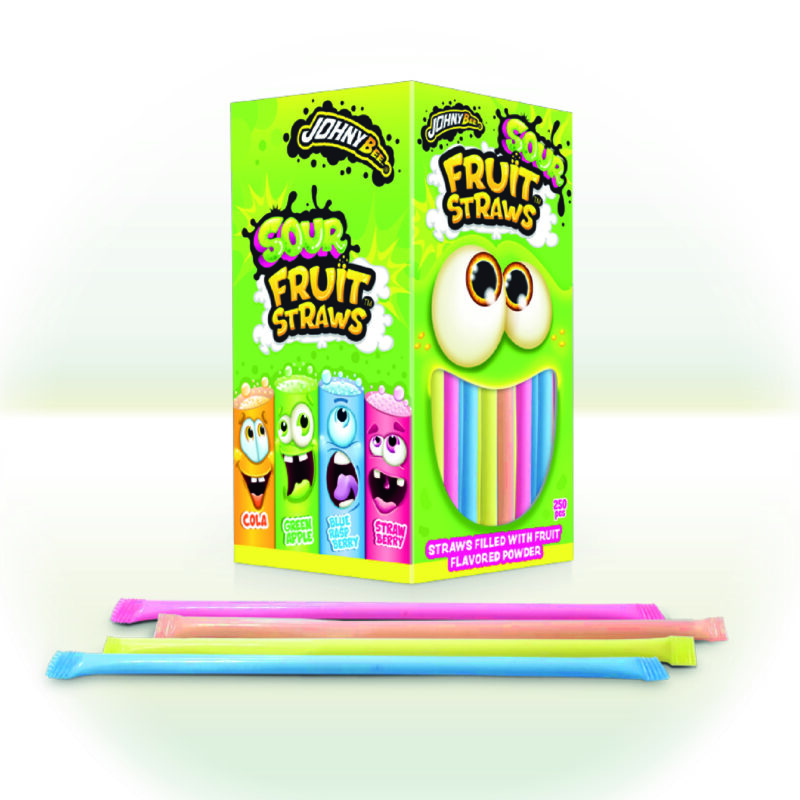The image is a rectangular illustration of a product mock-up for Johnny B. Sour Fruit Straws. The box, which has a vibrant lime green color, features four animated fruit straws with comical faces in orange, green, blue, and pink on its left side. The front of the box showcases a playful design with two large eyes and a mouth created from various colored fruit straws. The background comprises different shades of white and off-white, simulating a shiny surface, indicating that the product is placed on a counter or table. The product claims to contain 250 fruit straws in flavors such as cola, green apple, blue raspberry, and strawberry, all filled with fruit-flavored powder. In the foreground, there is a display of the four actual crimped and enclosed straws, representing the product's real-life appearance. The overall image is computer-generated without any real people or physical objects.